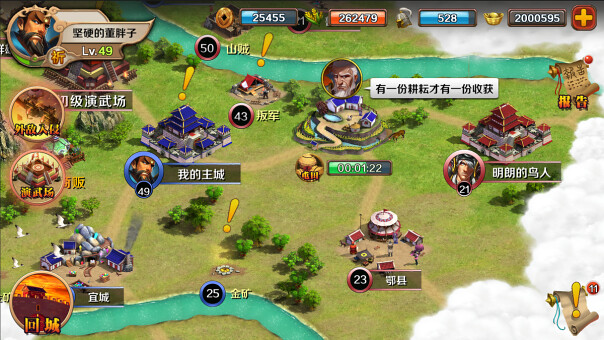The image resembles a vibrant video game screen, presenting a scenic view of green grasslands punctuated with sporadic yellow and brown patches, adding a natural yet cartoonish aesthetic. Amidst the greenery stand several structures, primarily temple-like buildings colored in red, blue, and brown hues. There are three prominent temples, one of which has a distinctive brown shade, setting it apart from the others. These structures are interconnected by a network of brown pathways, likely serving as routes for player navigation.

Bright yellow exclamation points hover over certain areas, likely marking points of interest or objectives within the game. The screen is adorned with detailed information panels on the left and top edges, showcasing a palette of oranges, blues, yellows, and reds. These panels include character portraits in circular frames, alongside detailed character information, icons, and numerical data, providing the player with crucial in-game insights and statistics.